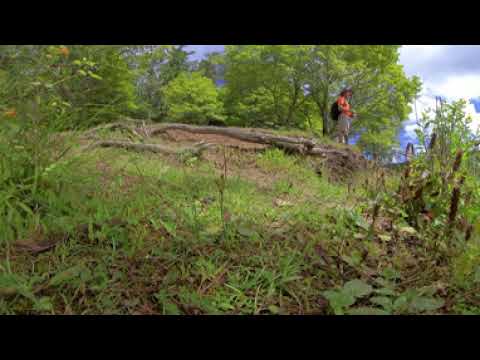The image captures a dynamic outdoor scene during the daytime, predominantly showcasing nature. A hiker, dressed in a peach-orange shirt, tan or white pants, and possibly wearing a hat, is centrally positioned, though they appear nearer to the top right of the frame. The hiker carries a black backpack and stands on a large fallen log that stretches across the center of the image, suggesting a recently cleared space within a dense forest. The foreground features various shades of green from the grass, shrubs, and weeds that are flourishing. In the background, a vast expanse of trees extends, enveloping the scene with rich, natural tones of green and brown. The sky above is a mix of blue, white, and gray, indicating a partly cloudy day. The image, framed with solid black borders at the top and bottom, gives a ground-level perspective, enhancing the height and scale of the surrounding wilderness. There is no text within the image, allowing for an immersive focus on the serene yet rugged natural environment.